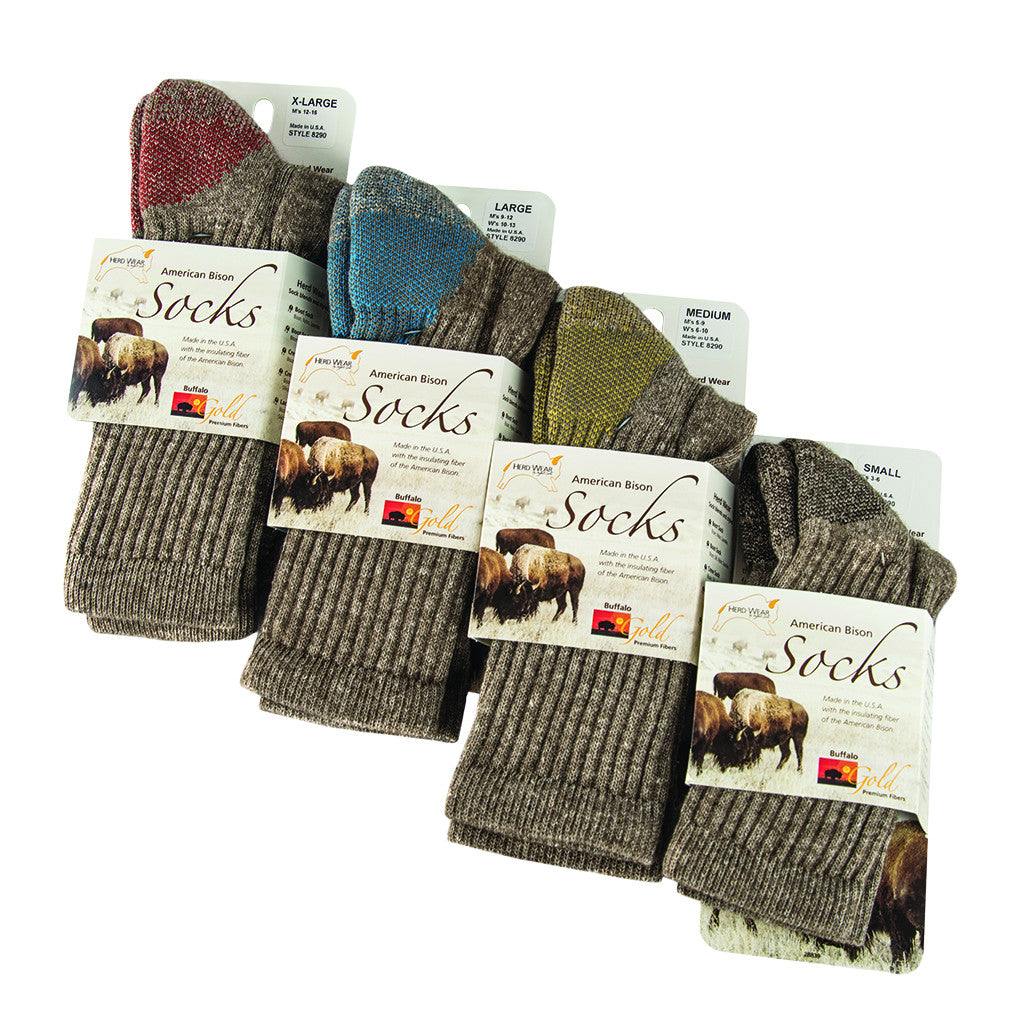This image showcases four pairs of American bison socks against a white background. Each pair is packaged with a tan label prominently displaying "American bison" in black at the top center, followed by the word "socks" in cursive. Below this is an image of a bison. Further down on the label, to the center-right, it reads "Buffalo Gold Premium Fibers" alongside a small red rectangle featuring a silhouette of a buffalo with a sun in the background. The socks themselves are predominantly brown or gray with color variations on the heel: one pair has a red heel, another blue, the third yellow, and the fourth black. Additionally, the socks are made in the USA using insulating fiber from the American bison, emphasizing their premium quality and unique construction from bison fur.